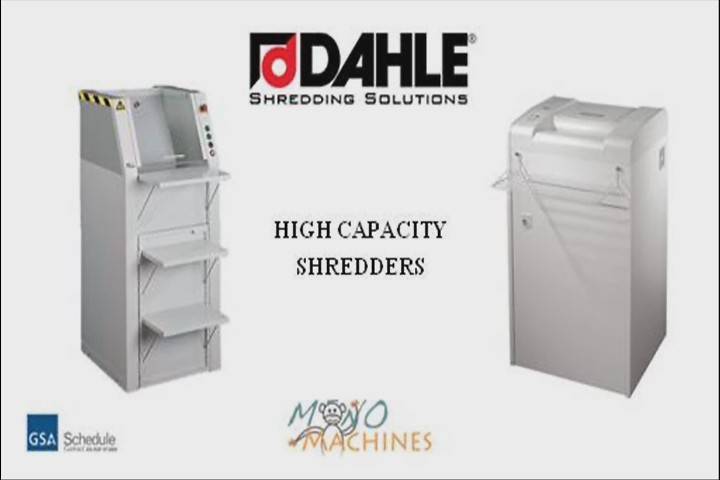This detailed color advertisement, likely sourced from a company magazine or brochure, showcases Dahle Shredding Solutions' high-capacity shredders available through Mono Machines. Featuring a completely white background, the ad prominently displays two sophisticated shredders. The first shredder on the left appears to be an advanced, high-capacity model with three distinct trays for sorting different types or sizes of paper. The second shredder on the right, more compact and boxy, resembles a photocopier with a top-loading slot. The Mono Machines logo includes a clever design where a monkey's head forms the first 'O' in "Mono," with the word "Mono" in green and "Machines" in yellow, while the rest of the text is in black. In the bottom left corner, a blue logo stamp with white lettering reads "GSA Schedule," adding a note of credibility. This advertisement effectively communicates the versatility and efficiency of Dahle's office shredding solutions aimed at high-capacity needs.